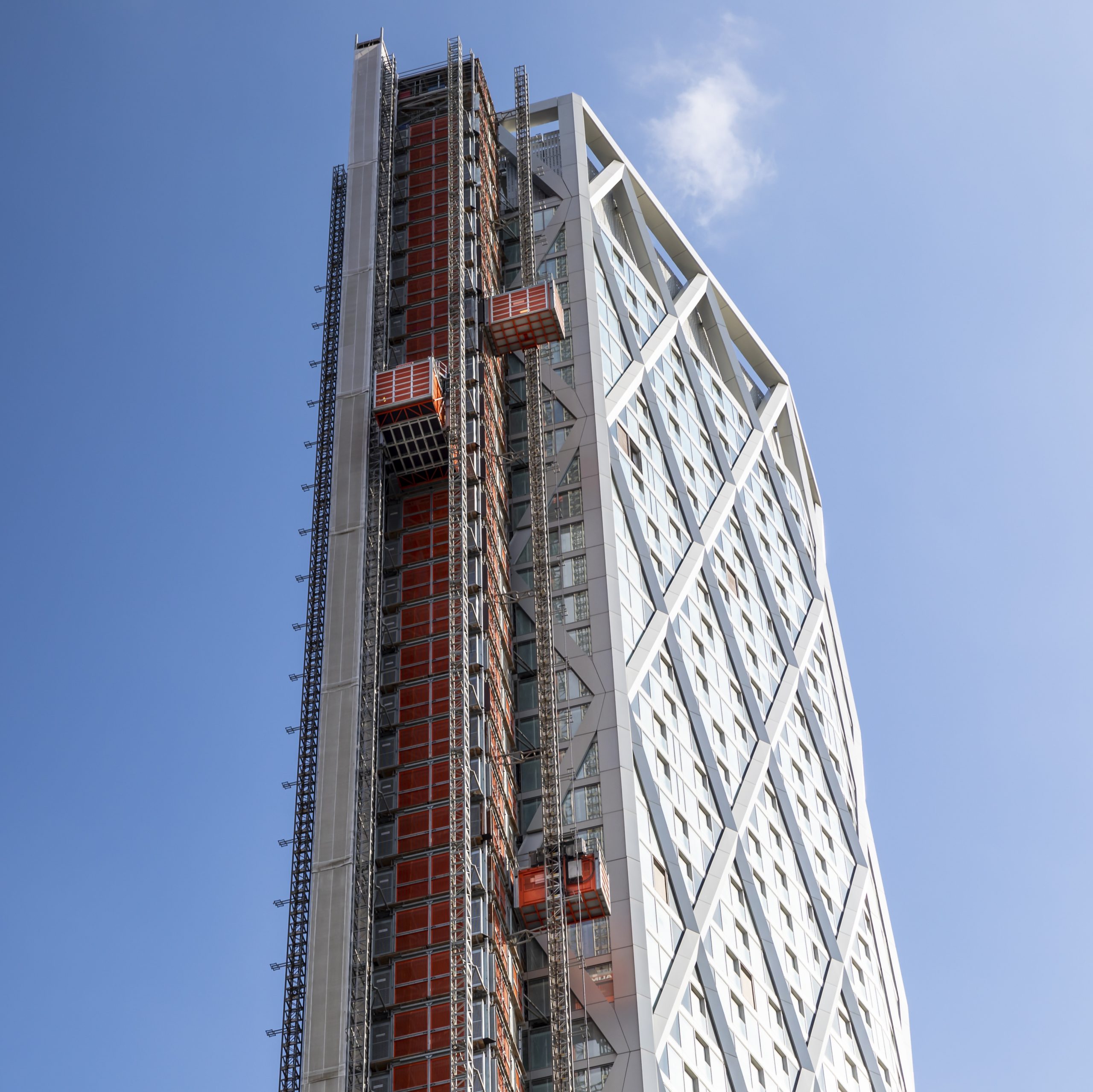The image showcases a high-rise building under construction, standing against a backdrop of a clear blue sky with one wispy cloud near the top. The building itself is predominantly white, featuring a crisscross diamond pattern formed by blue and white lines, and is adorned with numerous windows. On the left side of the building, there are three vertical access elevators with tracks resembling roller coaster rails, each characterized by red insides and silver outlines. These elevators, which appear to be used for transporting building materials rather than people, consist of open crates or cages—one red and brown box is visible ascending, while others are either stationed near the top or descending. The overall scene captures the dynamic process of construction against a serene skies.